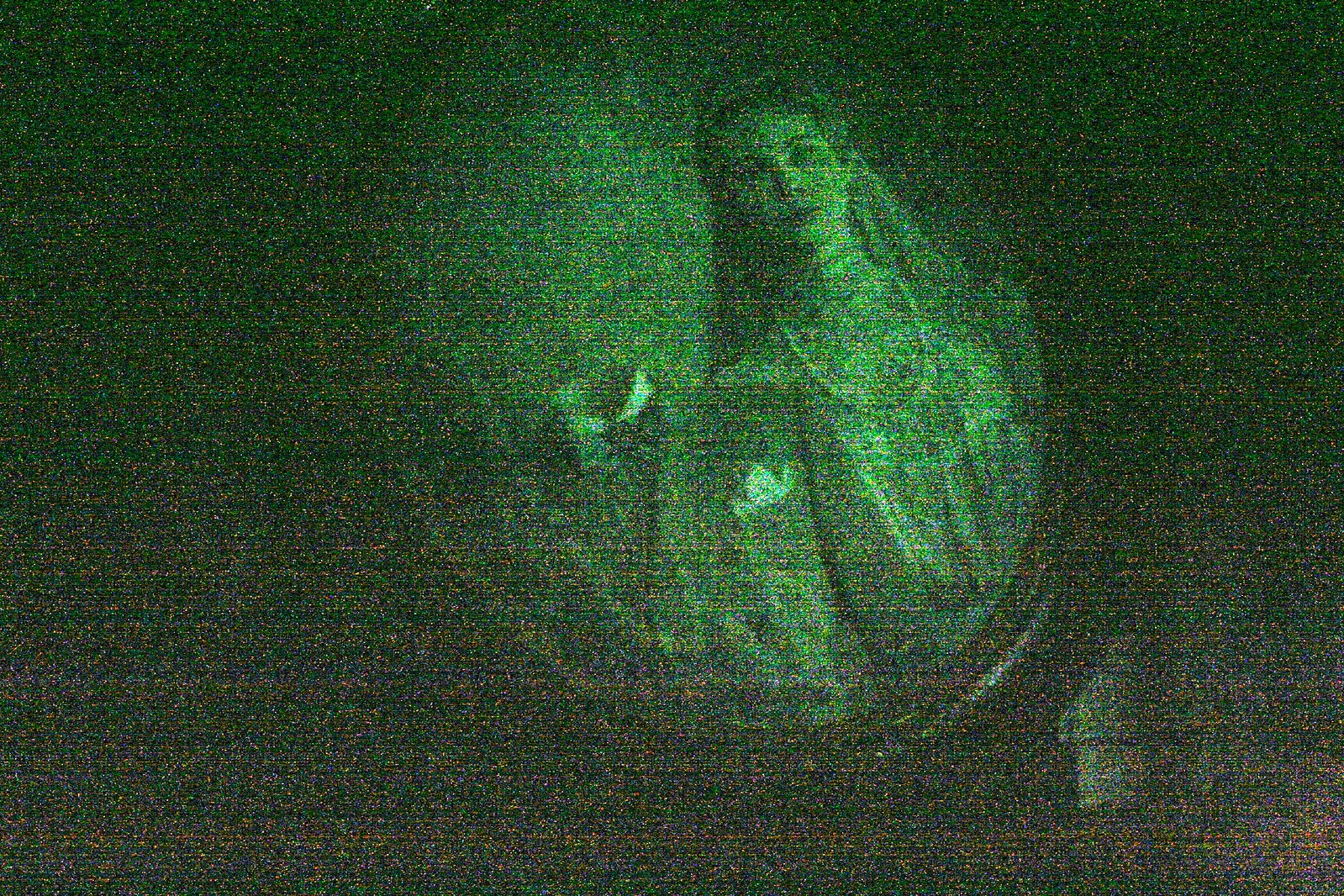In this night vision-like, grainy photograph, a dark and gloomy ambiance envelops the scene, reminiscent of a disturbed TV signal quality. Predominantly green, the image features scattered, grainy pinkish dots. Central to the picture is a faint, circular area where a white woman with long hair and a pearl necklace becomes visible. She stands in what looks like an old 1920s bedroom, peering into an antique mirror. Her attire seems to include a dress, though the details are blurred and distorted, making it difficult to discern more specifics about her exact pose or surroundings.